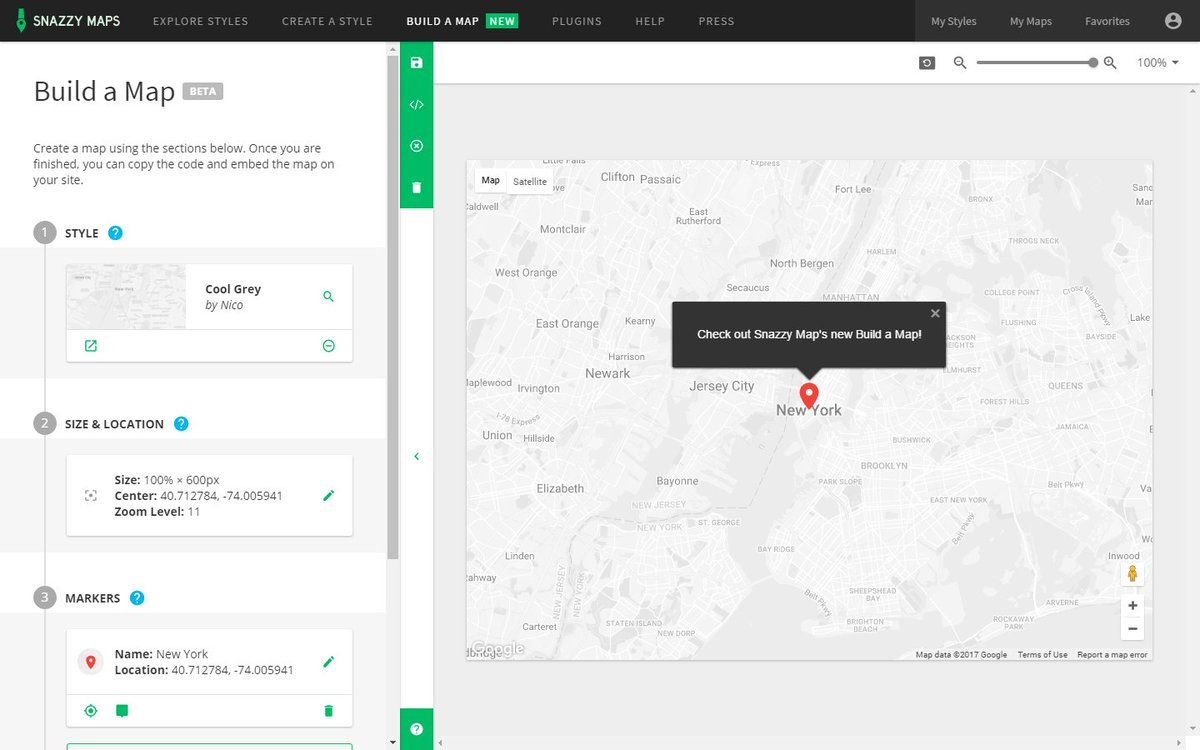The interface at the top displays several options, including "Snazzy Maps," "Explore Styles," "Create a Style," "Build a Map," "New," "Plugin," "Help," "Press," "My Style," "My Map," and "Favorites." 

On the left side, a section titled "Build a Map Beta" is present. It guides users to create a map using tools provided below, and mentions that once the map is complete, the code can be copied and embedded onto a website.

The interface includes a blue circle with a question mark labeled "Cool Gray" by Nico. 

Map dimensions are specified as 100% width by 600 pixels height, centered at coordinates 40.712784, -74.005941 with a zoom level of 11. 

Three markers are identified, with the first being New York, located at 40.712784, -74.005941. The map is displayed on the right side, featuring a red location pin in New York City. 

A final note reads: "Check out Snazzy Maps' new Build a Map."